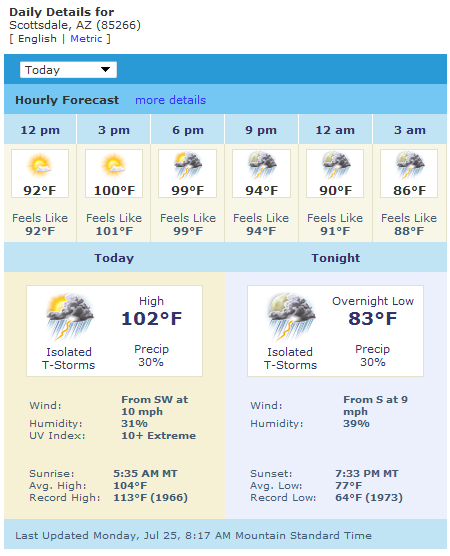In this screenshot taken from a weather website, we see detailed daily weather information for Scottsdale, Arizona, specifically for the zip code 85266. The interface offers both English and metric units, with the option to switch to metric via a hyperlink. 

At the top, a blue banner features a dropdown menu for selecting various days, currently set to "Today." Below that, a light blue banner provides an "Hourly Forecast," which can be accessed for more details through another blue hyperlink. 

The forecast is broken down by the hour: 

- **12 p.m.**: 92°F, feels like 92°F.
- **3 p.m.**: 100°F, feels like 101°F.
- **6 p.m.**: 99°F, feels like 99°F, with thunderstorms.
- **9 p.m.**: 94°F, feels like 94°F.
- **12 a.m.**: 90°F, feels like 91°F.
- **3 a.m.**: 86°F, feels like 88°F, with isolated thunderstorms.

Further down, a blue banner titled "Today and Tonight" provides additional summary information against a yellow background:

- **High**: 102°F, with isolated thunderstorms and a 30% chance of precipitation.
- **Overnight Low**: 83°F, with isolated thunderstorms.

This highly detailed weather layout visually communicates the forecast for various times throughout the day and night, highlighting temperature variations, perceived temperatures, and potential weather events like thunderstorms.